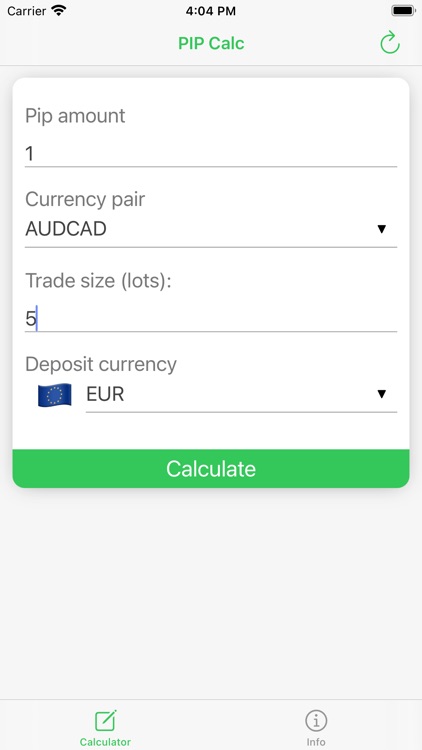This image appears to be a screenshot taken from a smartphone, displaying an application interface. At the top of the screen, a gray status bar shows the carrier information on the left, followed by a Wi-Fi symbol. Centered in this bar is the time, "4:04 PM." On the right side, there is a black battery icon. Beneath the time, a green label reads "PIP Calc" with "C-A-L-C" evidently indicating the app name. To the right, under the battery icon, is a C-shaped arrow symbol.

The main part of the screen is a white area with a series of labeled input fields. The first field is labeled "PIP amount," followed by an entry of the number "1." The next field down is labeled "Currency pair," filled in with "AUD/CAD." On the far right of this field is a black downward-pointing triangle, suggesting a dropdown selection for choosing different currency pairs. 

Below this, there's a field labeled "Trade size" with "Lots" in parentheses. This field shows the number "5," and there is a cursor placed next to this number indicating that this field is currently active for input. 

Further down, the label "Deposit currency" appears alongside a blue flag icon encircled by a ring of lights or dots. This is followed by the text "EUR - Euro." To the right of this, there is another black downward-pointing triangle for selecting a different currency. 

At the very bottom of the white area, a green bar spans the full width of the screen with the word "Calculate," suggesting a button that executes a calculation.

Beneath this white area, another gray section is visible, which is blank. At the absolute bottom of the image, two icons are present: one on the left that likely represents a calculator, colored green with the label "Calculator," and another on the right, a gray circle with an "i" inside, labeled "Info."